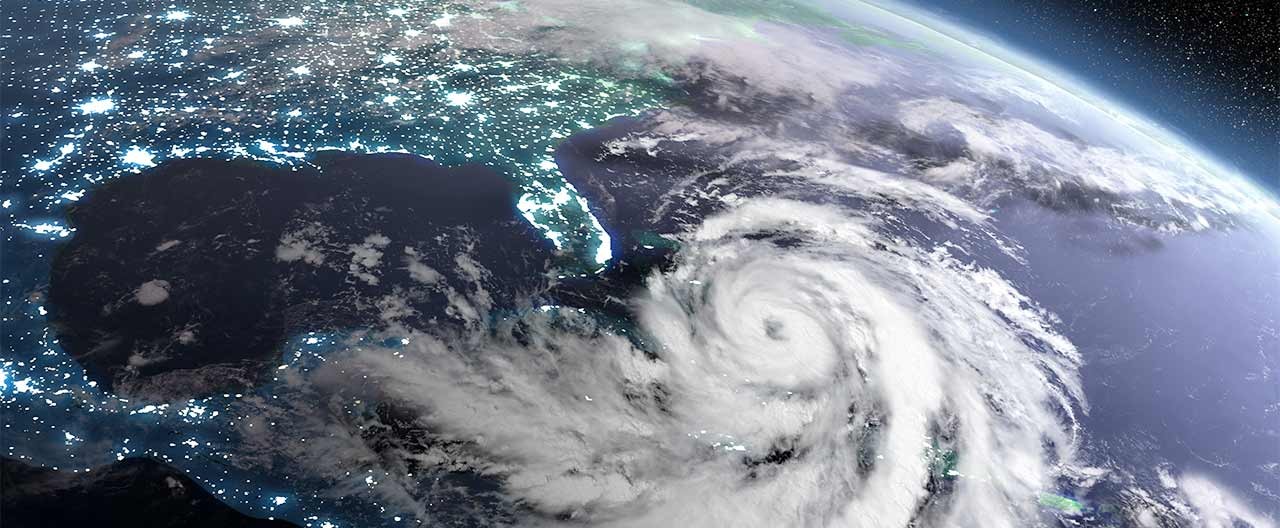This striking image, captured by a satellite orbiting Earth, presents a panoramic view encompassing parts of North and Central America, including the United States and the Mexican coast, extending into the Caribbean. The prominent Florida Peninsula is distinctly visible. Dominating nearly 40% of the lower right section of the image, a massive hurricane with its clearly defined eye and swirling white clouds commands attention. The terrestrial portions of the image, visible to the upper left and extending towards the bottom, are dotted with city lights, creating a greenish and bluish hue that outlines the population centers against the darker backdrop of the land. The oceans appear as deep blue expanses, contrasting with the landmasses. In the top middle section, purple clouds obscure parts of the land, while the upper right corner reveals the black expanse of space sprinkled with tiny white stars. This detailed and vibrant depiction underscores the dynamic interplay between land, sea, and atmospheric phenomena as viewed from space.